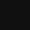The image features a large, solid black box, slightly smaller than an adjacent yellow box filled with intricate details. The black box appears empty and lacks any discernible features, starkly contrasting with the yellow box. Inside the yellow box, numerous small icons are arranged systematically, each associated with its respective bullet point. These icons include a mountain peak, a lightbulb, a sheet of paper with pencil writing, a thumbtack, a magnifying glass, and an ancient East Asian building. Additionally, a green circle is also present. The yellow box contains textual instructions guiding the viewer to carefully observe the image, scrutinize the objects and their quantities, discern the text, and note positions and subtle details. The black box’s minimalism juxtaposes the detailed, instruction-filled yellow box, highlighting the stark difference in content and purpose.